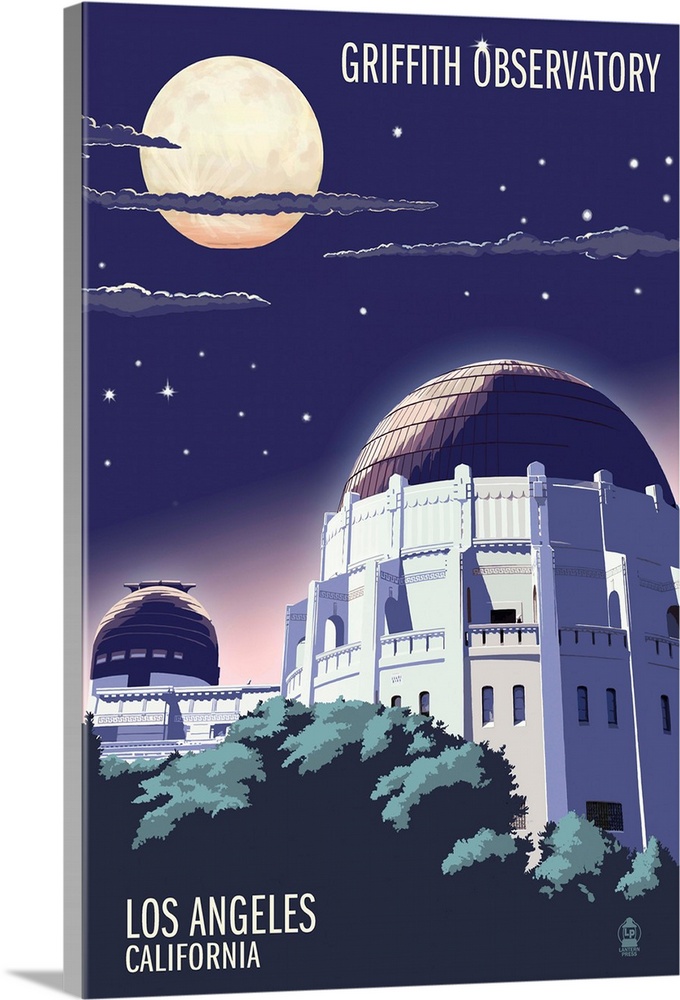This image is a highly detailed artistic rendering of the Griffith Observatory, presented on a three-dimensional canvas mock-up with a dark blue background. The central focus is a serene nighttime illustration featuring the observatory itself. The main building is a white, circular structure capped with a dome that appears to be a blend of brownish-beige and dark purple hues. To the left, there is a smaller, similarly designed observatory.

The sky above is adorned with glowing stars and wisps of gray clouds partially obscuring a bright full moon in the top left corner. The phrase “Griffith Observatory” is prominently displayed in bold, white letters at the top right, incorporating a star motif within the "O". The bottom left corner features dark green trees and the text "Los Angeles, California," grounding the scene in its real-world location.

Additionally, the bottom right corner includes the logo for Lantern Press, depicted as a lantern with the initials "LP" inside, adding a touch of authenticity and artistic branding to the piece. The entire image evokes a peaceful, nighttime atmosphere, making it suitable as a poster, billboard, or book cover celebrating the iconic observatory.